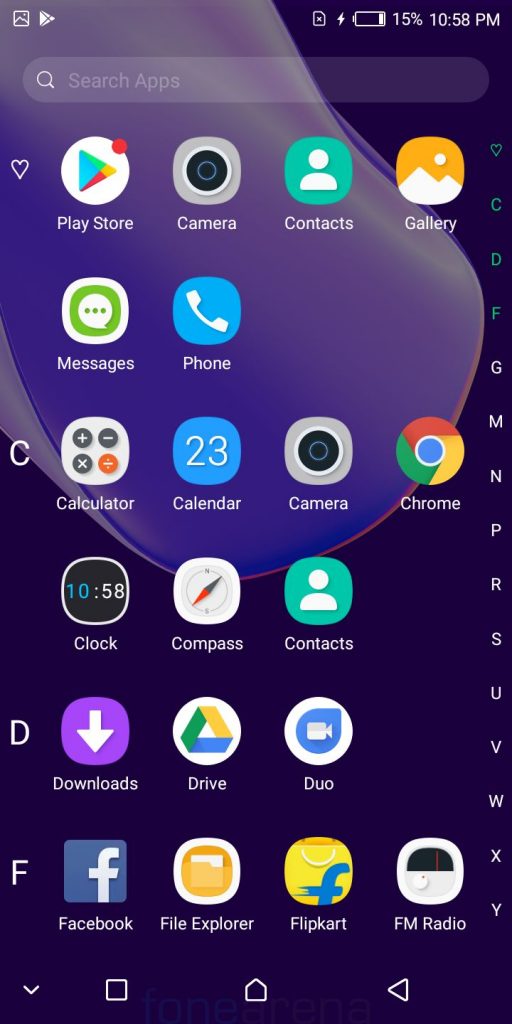The image displays a smartphone screen with an organized array of apps. At the very top of the screen, there's a status bar showing a square icon, the App Store icon, an unidentified icon, and a lightning bolt indicating the device is plugged in and charging, with the battery level at 15%. The time displayed is 10:58 PM. Below the status bar is a search bar with a magnifying glass icon, prompting users to "search apps."

On the left side of the screen, a vertical alphabetical list is visible, starting with segments labeled "HEART," "C," "D," and "F." This suggests the apps are categorized alphabetically. On the right side, smaller text lists letters from A to Z, indicating the alphabetical indexing of all installed apps. Notably, the letters corresponding to the sections currently visible on the screen (HEART, C, D, F) are highlighted in green, while the others are in white text.

Within the "HEART" section, the displayed apps include Play Store, Camera, Contacts, Gallery, Messages, and Phone. The "C" section lists Calculator, Calendar, Camera, Chrome, Clock, Compass, and Contacts. The "D" section includes Downloads, Drive, and Duo. Lastly, the "F" section shows Facebook, File Explorer, Flipkart, and FM Radio.